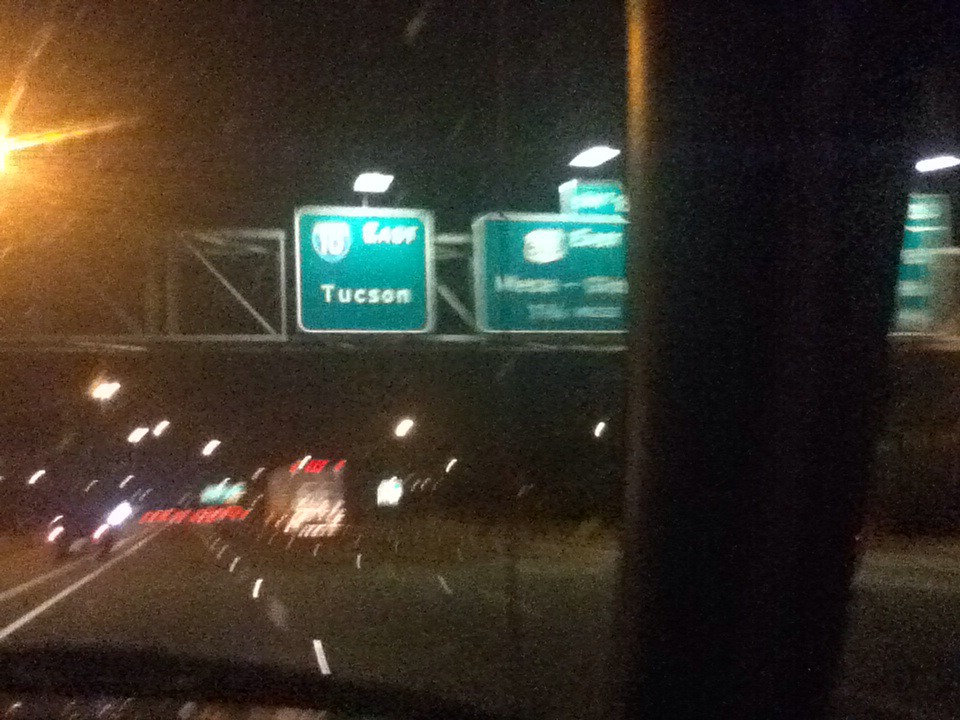A motion-blurred photograph captures a moment on a highway, as seen through the windshield of a moving vehicle. Prominent in the image are overhead green highway signs, typical of U.S. roads, suspended from a silver lattice structure and outlined in white. The signs, illuminated from above by bright lights to ensure visibility for drivers, include a notably clear one directing to "I-10 East Tucson," while the adjacent sign remains extremely blurry. A large beam from the car obstructs a significant portion of the right-hand side of the image. On the left, a warm golden glow from a light source creates a striking contrast. The distance reveals an array of red brake lights from numerous trucks and a prominent white truck, accompanied by a smaller, less distinguishable black vehicle. The overall darkness of the scene limits further detail, emphasizing the nighttime setting.